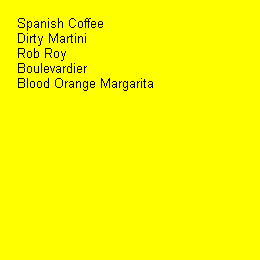The image is a small square with a solid bright yellow background and features black text, neatly aligned in the top left corner. The text, which appears pixelated and uses a regular font, lists the names of various drinks, each starting with a capitalized first letter followed by lowercase letters. The sequence of drink names, stacked one below the other, reads: Spanish Coffee, Dirty Martini, Rob Roy, Boulevardier, and Blood Orange Margarita. There are no other features or details in the image, making it seem like a simplistic, text-based snippet of a drink menu, possibly from a restaurant or bar.